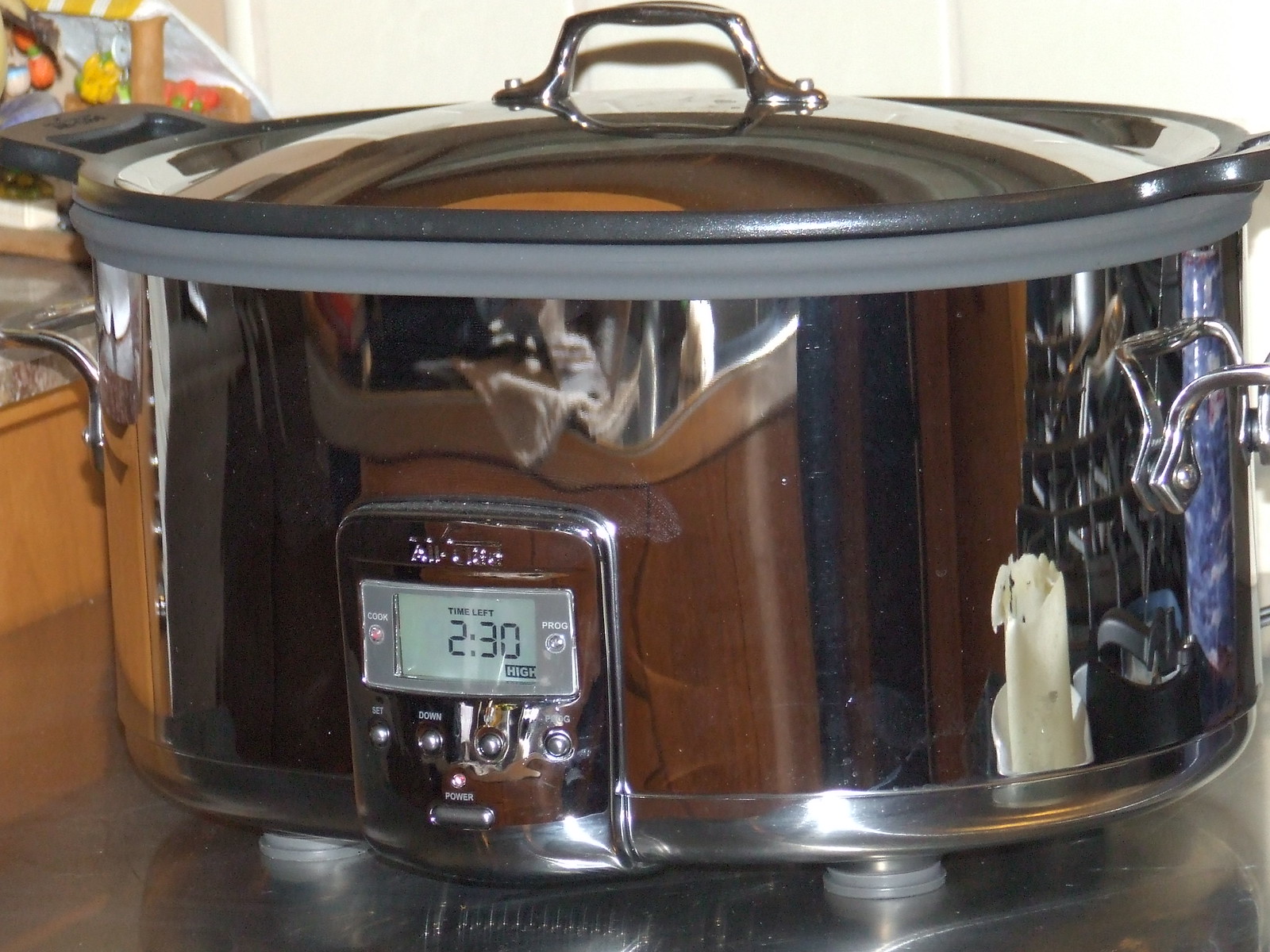The photograph is a detailed, close-up, color image of an oval-shaped stainless steel pressure cooker or crockpot, positioned in a kitchen setting. The highly reflective surface of the crockpot reveals various reflections, including a light source and a white candle, as well as the front edge of a worktop and the dark front of a kitchen cabinet behind the photographer. The tightly cropped image shows the lid of the pot with a top handle, and partial views of the side carrying handles. In the foreground, two grey plastic or rubber circular feet are visible. Prominently displayed on the front of the crockpot is an LCD screen indicating "2:30," potentially representing either 2 hours and 30 minutes or 2 minutes and 30 seconds remaining on a timer. Silver control buttons are situated beneath the screen, with various settings including off, slow, low, high, and possibly a warm function, with the power light illuminated, suggesting the device is in operation. The cooker sits atop a probable kitchen counter, and to the left, blurred objects are hinted at on the counter behind, adding context to the domestic environment.